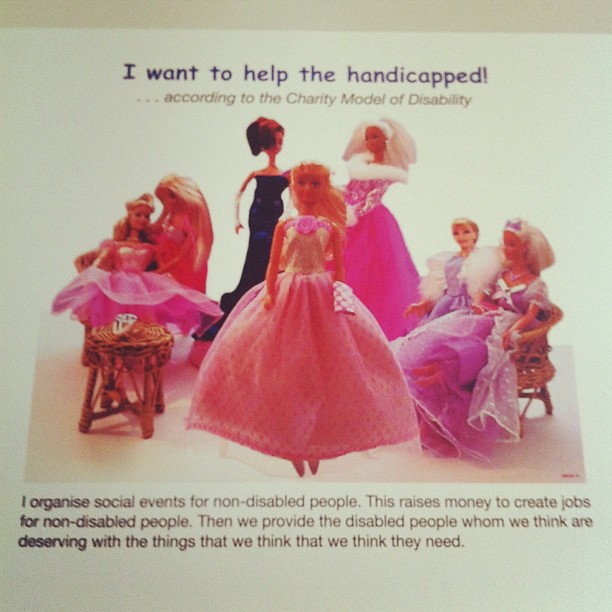The image in question appears to be a satirical poster critiquing the charity model of disability. At the top, it prominently features the text, "I want to help the handicapped..." followed by "according to the charity model of disability." Below this, there is a large, composite photograph of numerous Barbie dolls, primarily dressed in pink dresses, with a few wearing variations like a purple dress and one in a black dress. Some of these dolls are seated, while others are standing, creating a collage-like effect. Beneath the photo, the text reads, "I organize social events for non-disabled people. This raises money to create jobs for non-disabled people. Then we provide the disabled people whom we think are deserving with the things that we think they need." The use of Barbie dolls, frequently associated with a certain demographic, seems to emphasize the critique of out-of-touch charity approaches by depicting a superficial representation of support for disabled people.